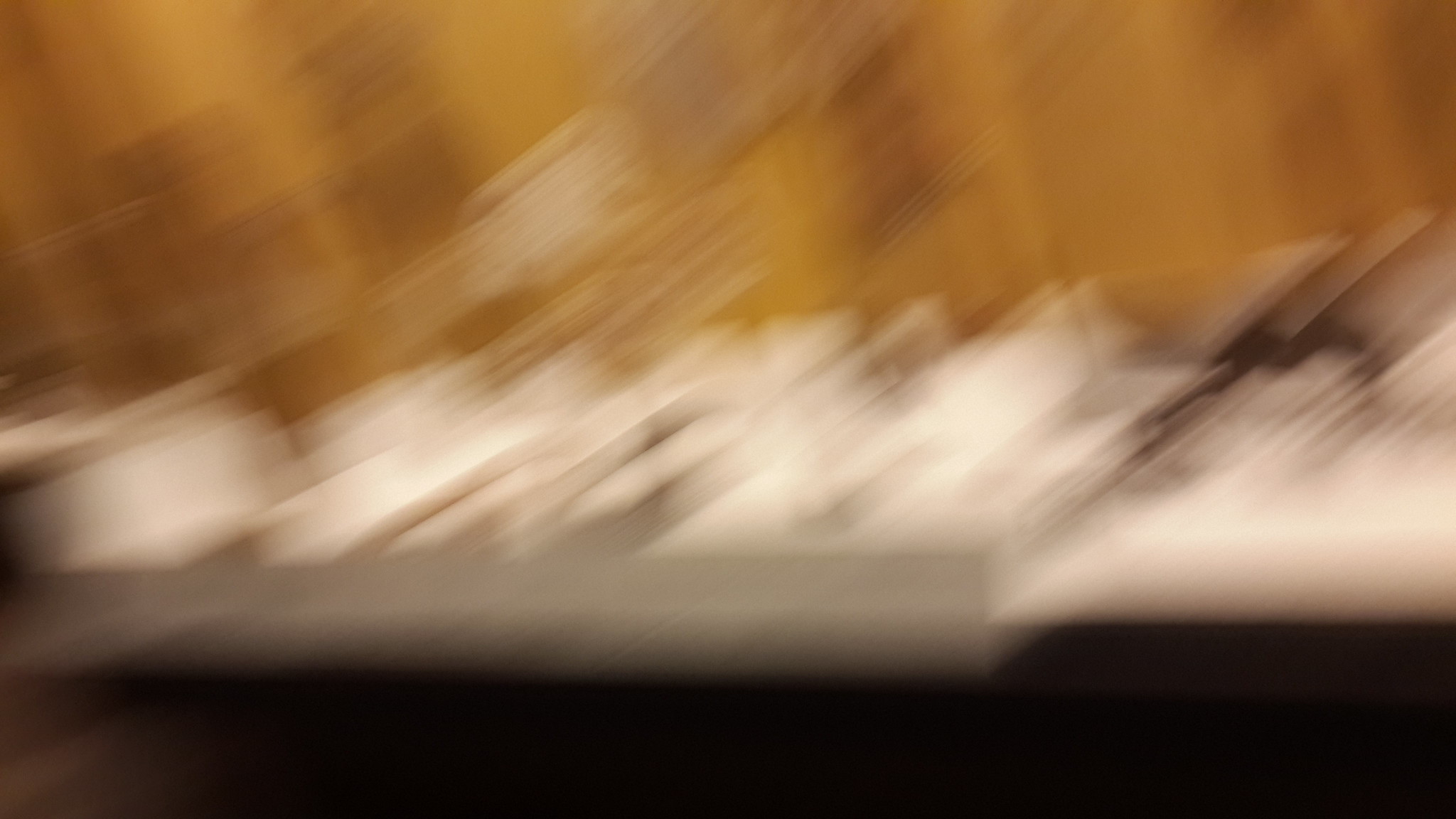This extremely blurry photograph primarily depicts a long rectangle divided into distinct color regions. At the top, there is a blend of an orange-brown hue, which could potentially resemble a brown wall. Below this section, occupying the middle of the image, there is a white blur that includes what appear to be diagonal white lines or objects against a gray shelf-like background. Some parts of these white elements are slightly darkened. Extending diagonally from the top right to the bottom left, the blurred lines within this area accentuate the sense of motion or distortion. Towards the bottom of the photograph, there is a shadowy, blackish-brown region that transitions into a darker area with a subtle hint of lighter color on the bottom left, potentially representing shadows beneath the shelf-like formation. Overall, the image lacks clarity, leaving the objects and their arrangement indistinct.